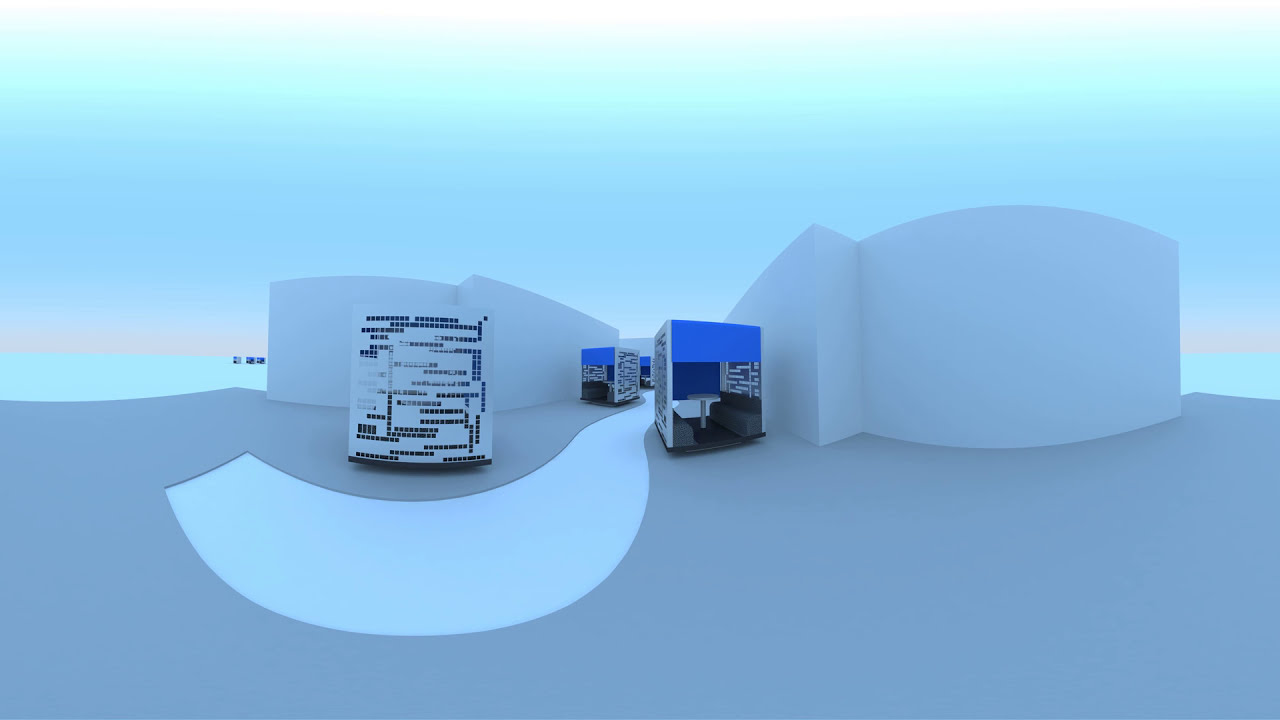This digitally rendered image depicts a futuristic, computer-generated landscape. At the foreground, there is a bluish-gray solid surface, possibly representing a modern, curvilinear roadway. Central to the image are four cubicle-like modules designed to resemble futuristic bench-style seating with small tables in between, evoking the appearance of a sophisticated, modern meeting area or dining space. These structures are reminiscent of modular computer chips with square cutouts and feature a curvy walkway weaving between them. The modules are set against wavy concrete structures, contributing to the modern aesthetic. The gradient background transitions smoothly from pastel blues to greens, becoming lighter and merging into a sky-like upper section. The detailed and varied hues include shades of blue, gray, white, black, brown, and orange, enhancing the complexity and visual appeal of the scene.